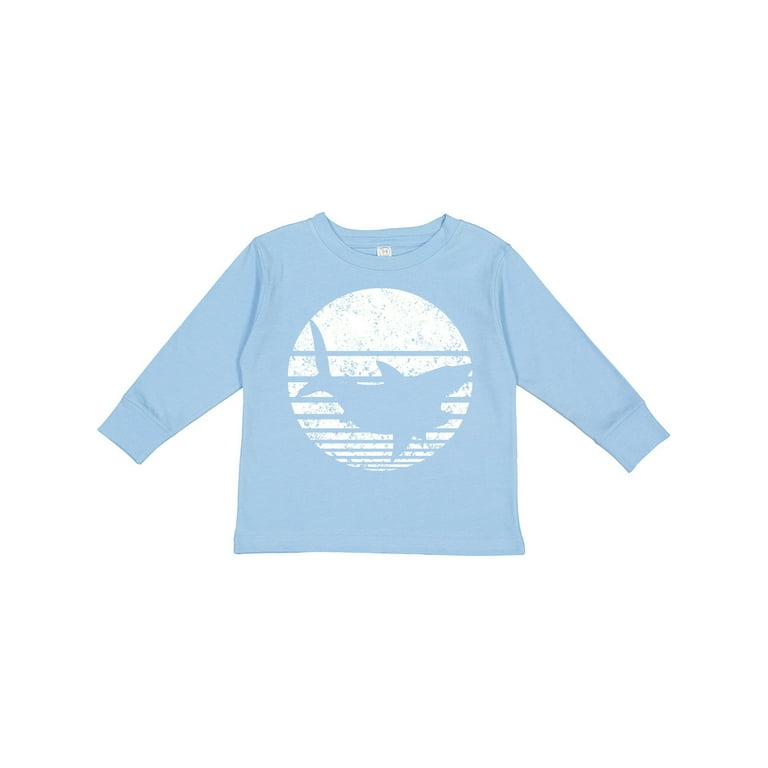This image portrays a long-sleeved, light blue child's shirt displayed against a white background. The shirt features a white manufacturer's tag at the back of the neck. Central to the design on the front of the shirt is a large, distressed white circle dotted with speckles of the light blue fabric, giving it a less opaque appearance. Across the circle, horizontal lines vary in proximity, closer together at the bottom and gradually spacing out towards the top. Dominating the bottom half of the circle is a light blue silhouette of a shark with an open mouth, a dorsal fin, pectoral fins, and a split tail fin, all in the same hue as the shirt. The shark's body is curved, creating an impression of motion as if it is swimming. The shirt has cuffs at the sleeves and a crewneck, indicating it's designed as a crewneck sweatshirt.